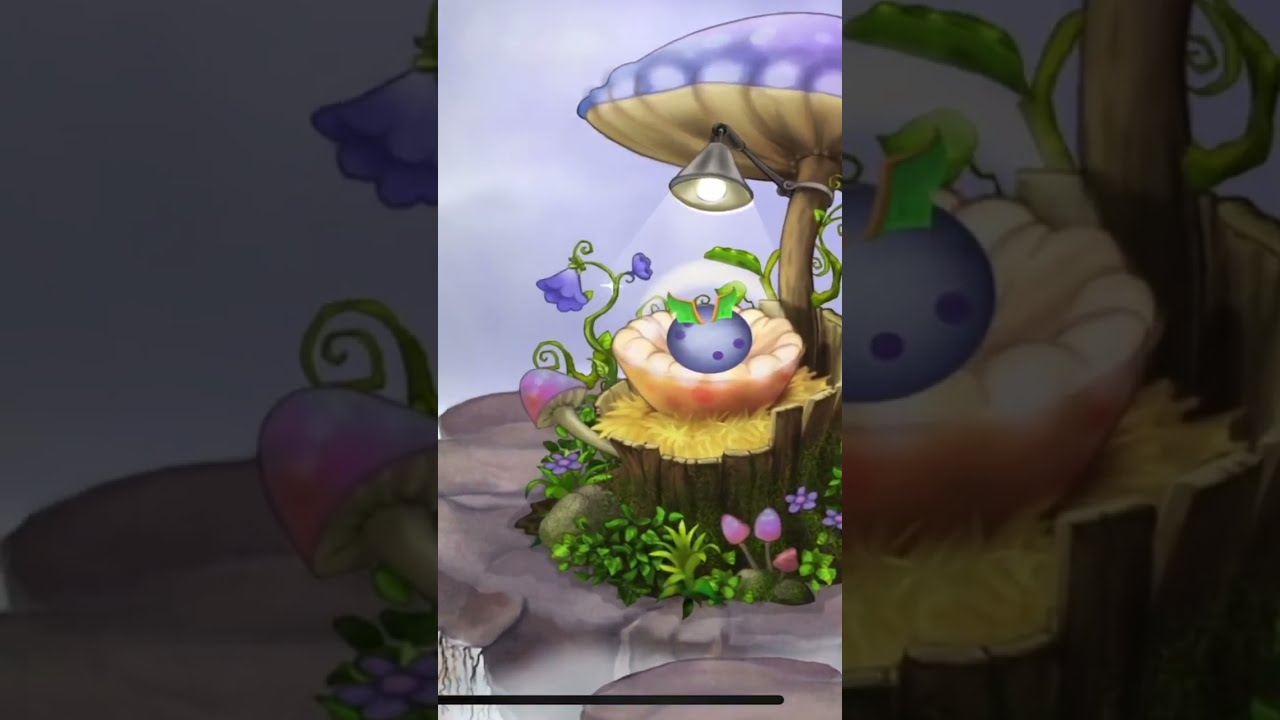The image is a whimsical, fantasy-themed cartoon drawing featuring a large, purple-topped mushroom with a tan stalk, which serves as the centerpiece. The mushroom has a lantern attached to its underside, casting a warm light onto a purple egg with darker purple dots nestled below. The egg rests inside a white, pillow-like basket, which sits atop a yellow, feathery bed inside a circular nest made of wood planks on a tree stump. The stump is placed on a large gray rock surrounded by an enchanting array of flora, including pink and purple flowers, green bushes, and additional small mushrooms. The background is a soft, light purple cloudy cover that emphasizes the focal elements. Interestingly, the background also features a repeated, zoomed-in, and darkened version of the main image, creating a layered, artistic effect.